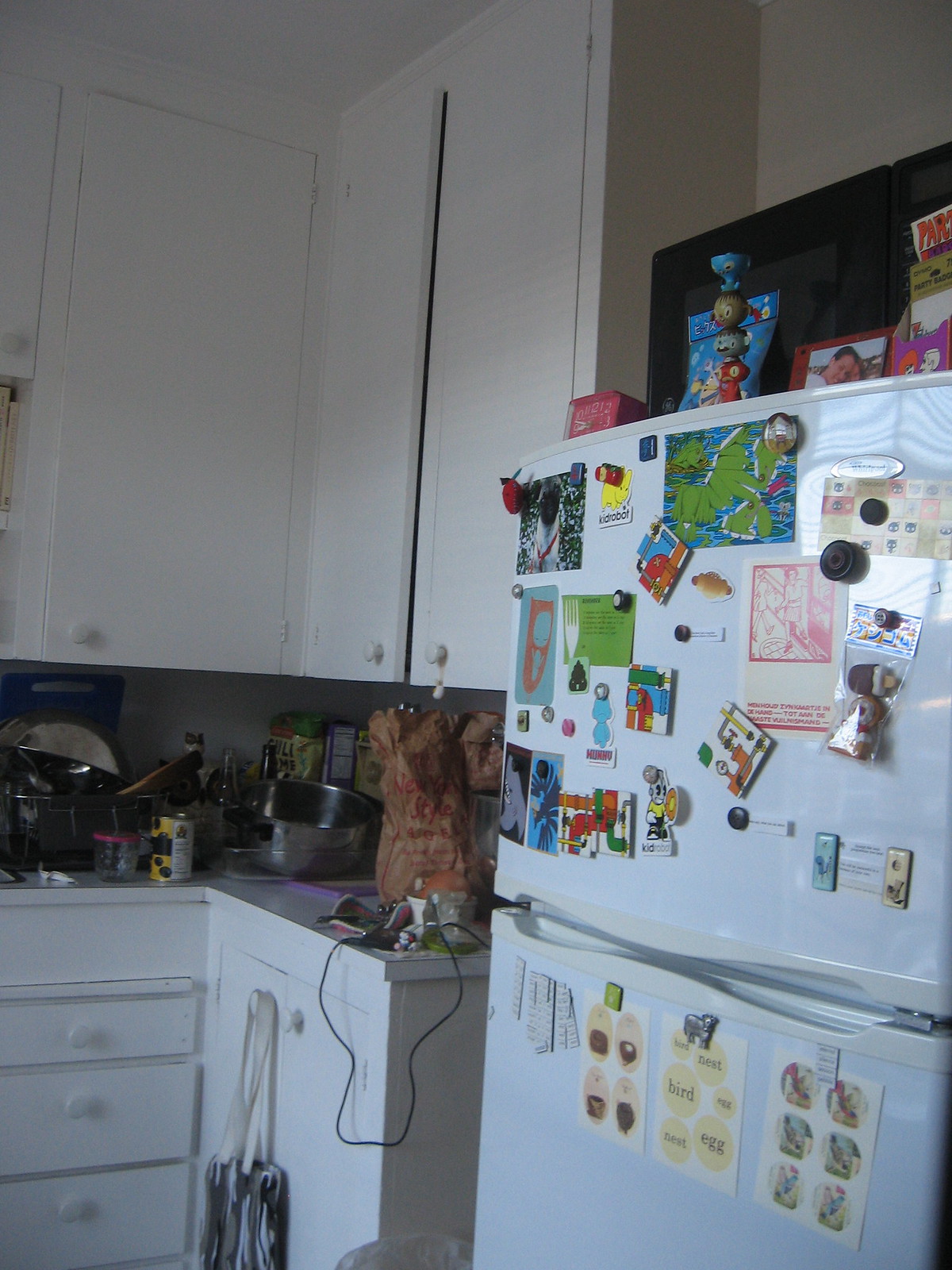The photo captures a detailed view of a kitchen corner. Dominating the scene is a white refrigerator with a top freezer and a bottom fridge, its surface adorned with an assortment of magnets and stickers. Among the magnets, there is a noticeable picture of a pug, and beneath it, a series of small postcards labeled "bird nest," "egg nest," and "egg," featuring images of eggs. Atop the fridge, a photo of a woman is displayed, accompanied by what appears to be egg holders or a small statue.

To the left of the refrigerator, white cupboards line the wall, each fitted with small round knobs at the bottoms of the doors. These cupboards mark the junction of the kitchen's corner. Below them, the white countertops match the cabinetry and are cluttered with various items. A fast food bag sits among the chaos, alongside a silver bowl with black handles. A tote bag hangs off one of the drawer knobs, near a visible cord. A dish rack, containing a blue cutting board and assorted dishes, adds to the busy scene on the counter. The overall impression is one of a well-used and personalized kitchen space.